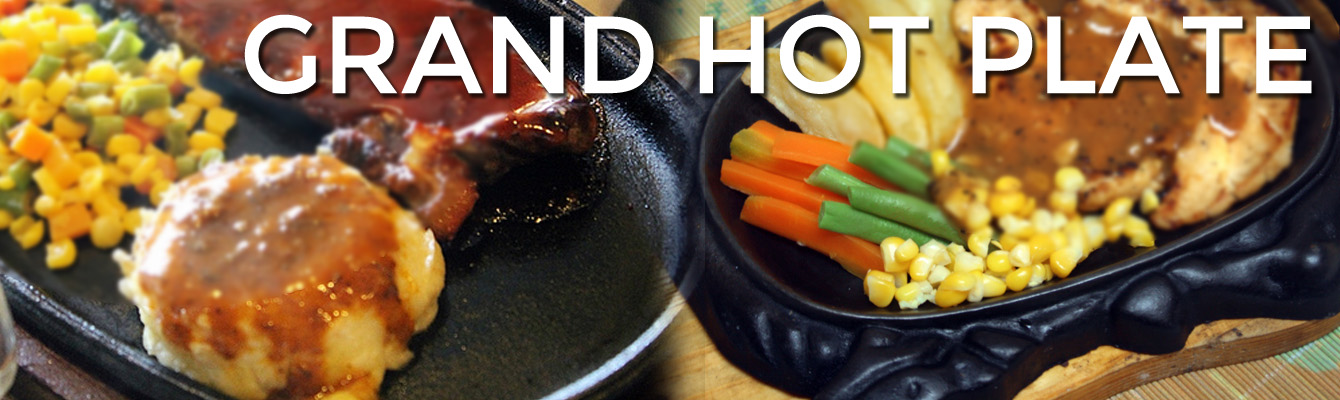The image showcases two black cast iron plates filled with a variety of foods, under the heading "Grand Hot Plate" in bold white text at the top. The plate on the left, set against a wooden surface, features mashed potatoes with gravy, a mix of corn, green beans, and chunks of carrots, and a serving of meat likely covered in barbecue sauce, possibly ribs. To the right, another black metal plate presents longer green beans, carrots, corn kernels, and a lighter piece of meat, potentially chicken with brown gravy. Additionally, this plate includes what seems to be lighter-colored fruit, perhaps pears. The vibrant colors of the vegetables—yellow from the corn, orange from the carrots, and green from the beans—contrast against the earthy tones of the meat and gravy, suggesting an appetizing and hearty meal. This image appears to be used in an advertisement, possibly for a restaurant, emphasizing its special offerings.